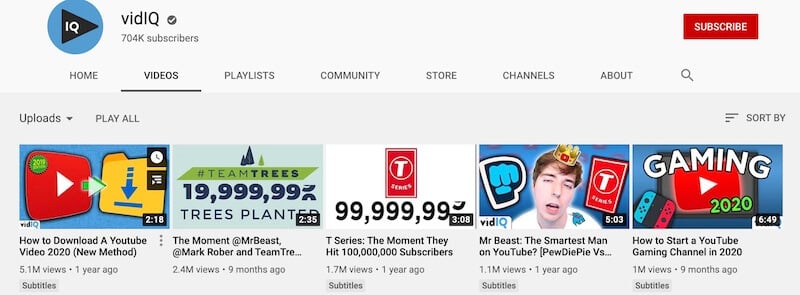This image is a screenshot from a video-sharing site similar to YouTube, featuring a clean, organized layout. The top header contains the company name, "VidIQ," where "vid" is in lowercase letters and "IQ" is in uppercase letters. The company's logo, a blue circle with a right-pointing triangle, houses the "IQ" written in white within the triangle. 

Beneath the header, a navigation menu stretches from left to right with links titled: Home, Videos, Playlist, Community, Store, Channels, and About. On the far right of the header is a search icon. 

The background color of the main content area is gray, and prominently displayed are five video thumbnails. Under a section titled "Uploads" with a "Play All" option, the thumbnails each feature a title and static image. The first video on the left is titled "How to Download a YouTube Video 2020 (New Method)." Adjacent to this, the second video’s title reads, "The Moment at MrBeast, Mark Rober at Team Tree," highlighting 19,999 trees planted. Each thumbnail and title hints at a diverse array of video content available on the site.